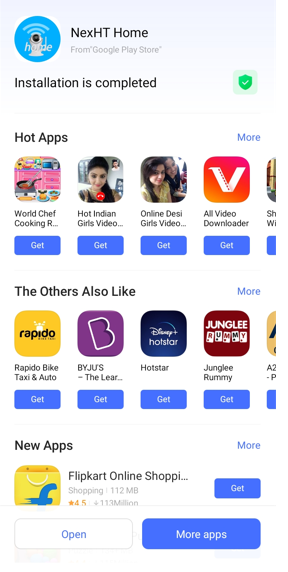Screenshot of a mobile app showing installation confirmation and popular app suggestions:

The screenshot showcases a mobile app with a clean, white background. At the top, there's a blue logo resembling a Wi-Fi signal beaming upwards. Adjacent to the logo, the title "Next HT Home" is prominently displayed in bold text. Directly beneath, in gray font, it reads "from Google Play Store."

The main section of the screenshot alerts the user that the "installation is completed," marked by a green checkbox beside this notification, emphasizing a successful app installation. Below this notification, a list of popular apps is displayed with their titles:

1. **World Chef Cooking**
2. **Hot Indian Girls**
3. **Online Desi Girls**
4. **Alt Video Downloader**
5. **Repto**
6. **Bike, Taxi and Auto**
7. **Byjus**
8. **Hotstar**
9. **Jungle Rummy**

Each of these apps features a blue "Get" button in white text, inviting the user to download them.

The image effectively highlights the app store interface, detailing the apps available for download and signaling completed installation, all set against a minimalist design background.